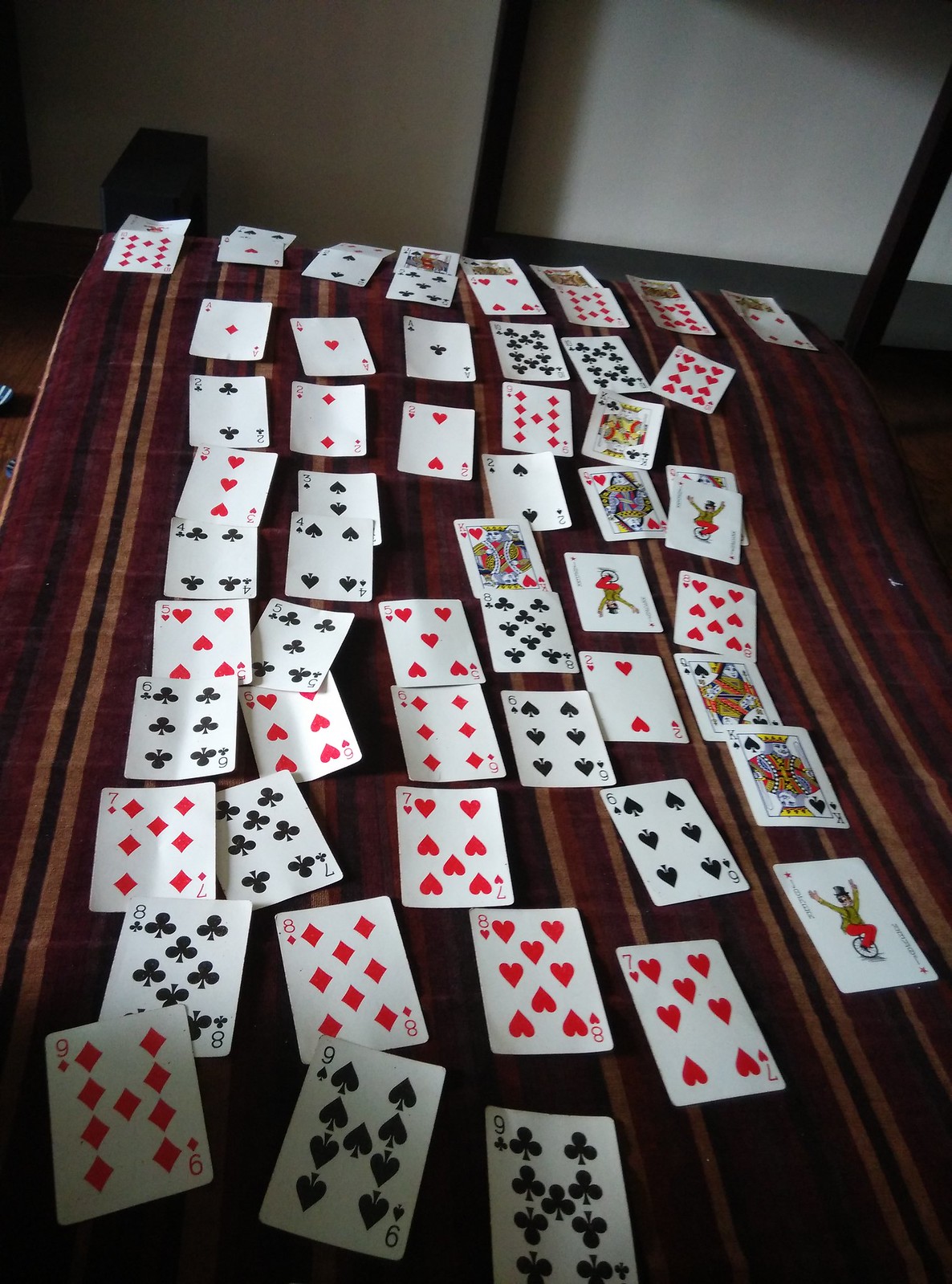The photograph showcases a spread of playing cards meticulously arranged on a bedspread adorned with brown, black, and gold stripes. The cards are sorted in numerical order, from nines down to sevens, though there appear to be some missing cards, hinting at an incomplete deck. Additionally, there are at least three jokers present, suggesting the use of multiple decks. The kings are unevenly distributed among the spread. Notably, several of the cards exhibit a distinctive bend at the center, likely indicating frequent use and manipulation by their owner who bends them for better concealment during gameplay.